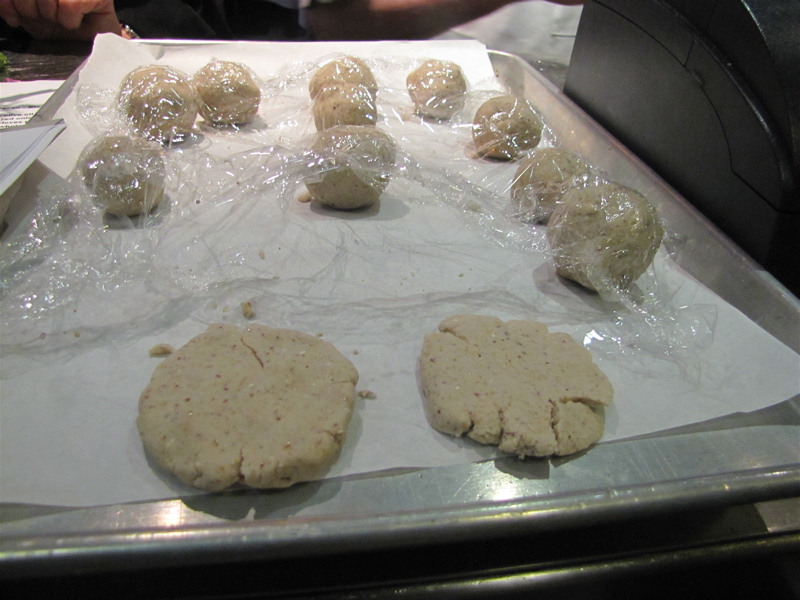In this image, we have ten balls of light white and light brown dough arranged on a large silver metal cooking pan. The dough balls, appearing to be cookie dough, are partially covered with wrinkled cling film, indicative of refrigeration. Most of them rest on white parchment paper, while two in the front, which have been flattened and show slight cracking at the edges, sit outside the parchment paper, ready for baking. To the right of the metal tray, there is a black partition, possibly a plastic wall or computer monitor tower. To the left, leaning against the tray, is a white booklet or notepad. The preparation scene is set for baking, suggesting these are likely sugar or molasses cookies.